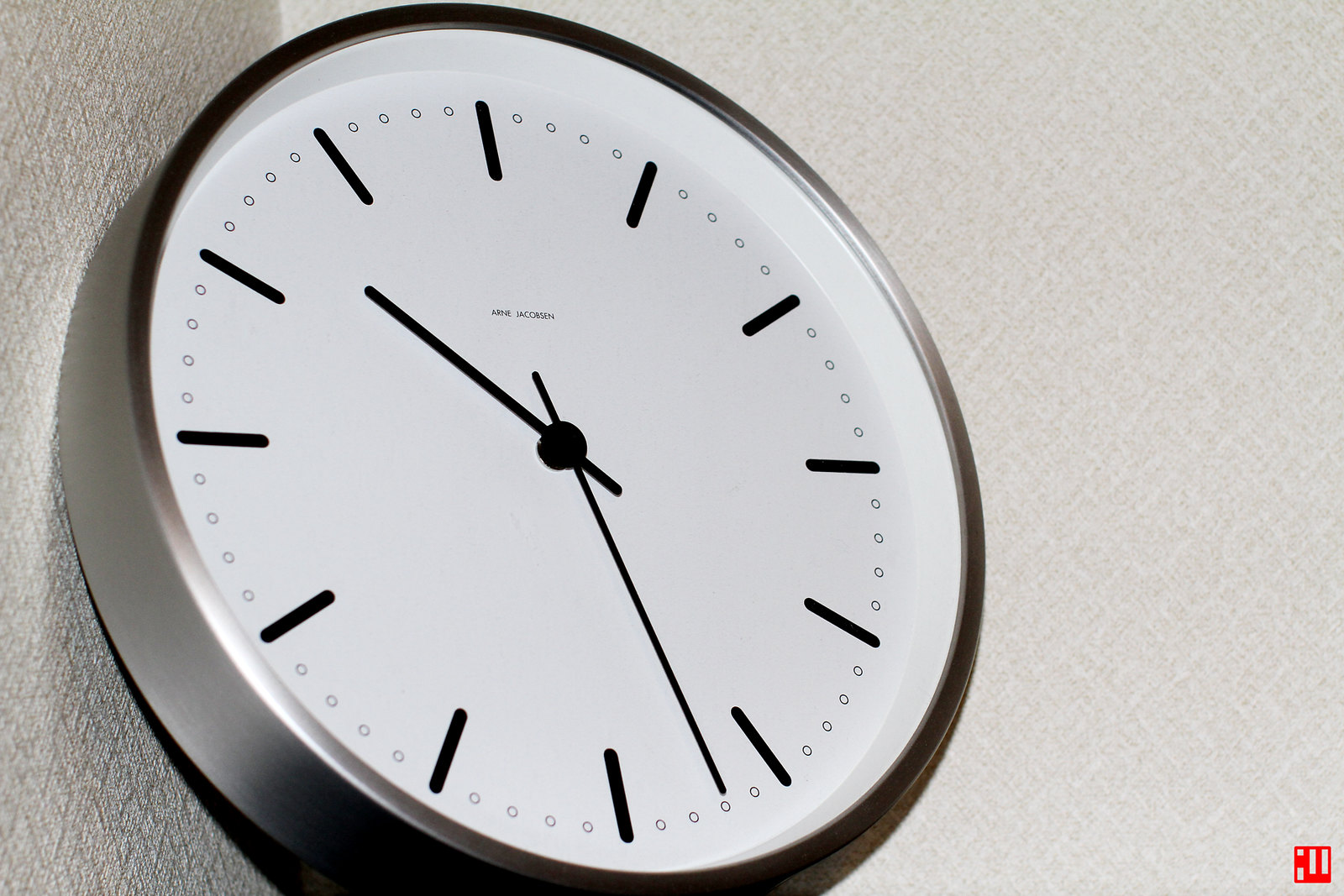In this image, a circular wall clock is prominently featured against a dual-toned wall. The clock's face is bordered with a sleek, silver rim and has a pristine white background. Instead of traditional numerals, the hours are marked by small, black lines. The clock hands, which are thin and black, contrast sharply against the white face. Adjacent to these hour markers are tiny circles that denote the seconds. The clock is positioned towards the left side of the composition, angled forward towards the right corner of the image. The wall behind the clock has two distinct shades; a dark gray on the left and a light gray on the right. In the center of the clock's face, there is a small, black inscription indicating its brand, which is too minute to decipher.